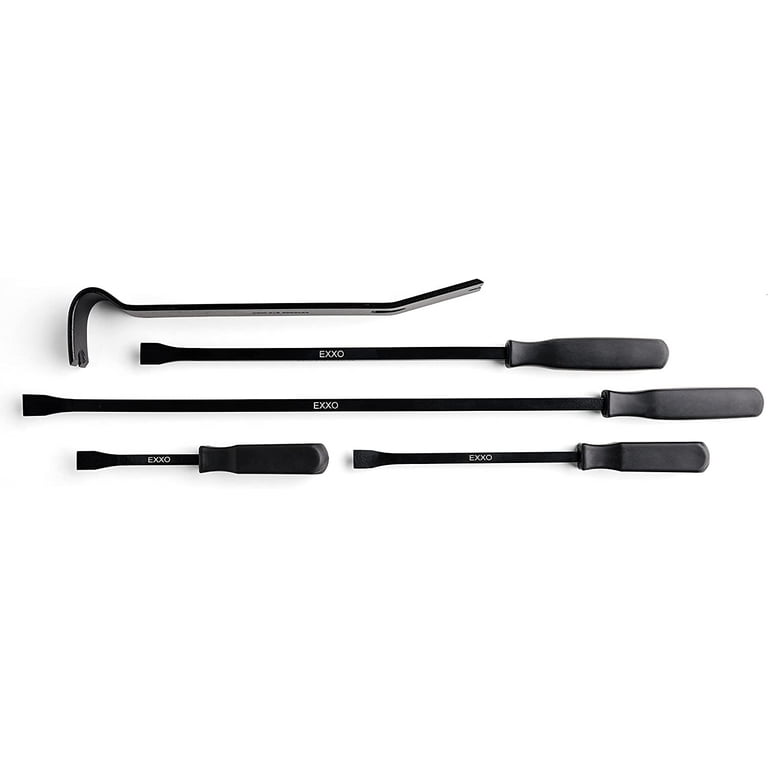The image features a five-piece tool set from the brand EXXO, all placed on a white background. Four of the tools resemble screwdrivers with flat-head designs, differing only in size. Each of these four tools has a grippy black handle, a long, skinny black shaft, and bold white uppercase "EXXO" lettering printed on the shaft. The sizes range from a very short one to a very long one. The fifth tool is distinct, featuring a hook-like design, which gives it a more specialized function, possibly for prying or pulling out nails or bolts. Unlike the other four, this hook tool does not have a handle but is similarly entirely black, with some indecipherable text tilted on its side.